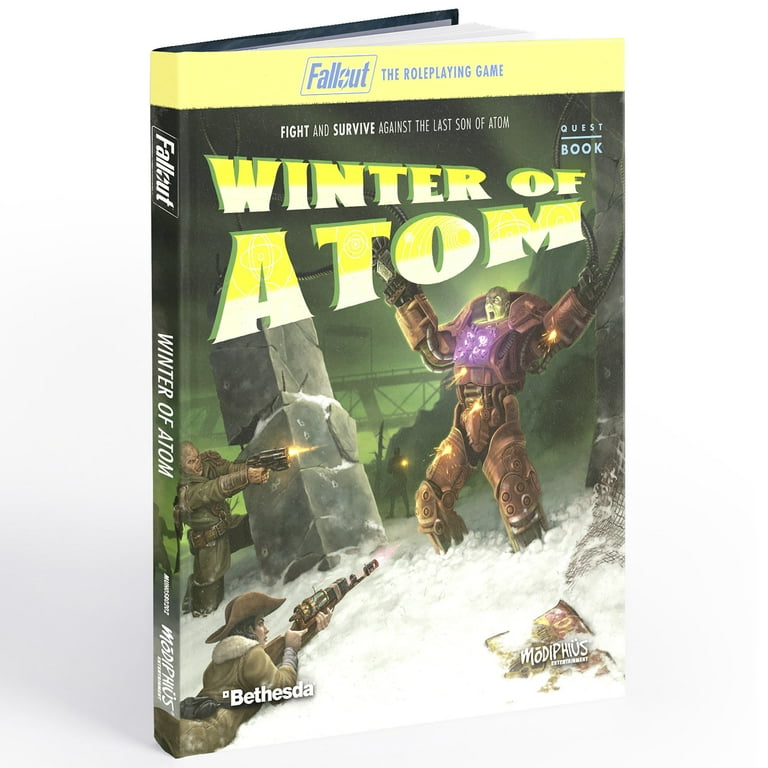This image shows a hardback book standing vertically on an isolated white background. The top of the book cover features a bright yellow band with italicized blue text reading "Fallout," followed by "THE ROLE-PLAYING GAME" in regular block caps. Below this, the cover illustrates a dramatic combat scene set against a grayish-green backdrop. In the lower left corner, a soldier lies on a snow-covered ground, aiming his rifle at a towering, heavily armored figure, possibly a robot or monster, depicted in the upper right. Surrounding the scene are tall, slate rock formations. Emerging from the left side of one of these formations, another soldier is visible. The scene involves men of various eras and genres, with one soldier appearing to wield a 1920s-style weapon and another armed with a futuristic gun, both aiming at what seems to be a Transformer-like adversary.

The title "Winter of Atom" is boldly written in yellow at the center of the cover; "Winter of" is in smaller text above "Atom." In the upper right corner, text reads "QUEST BOOK," underlined for emphasis. The lower left of the cover displays white text over the body of the soldier, reading "Bethesda." The spine of the book, shown on the left, vertically reads "Fallout," followed by the book's title "Winter of Atom" in white text. Below the title on the spine, additional white text reads "Modiphius."